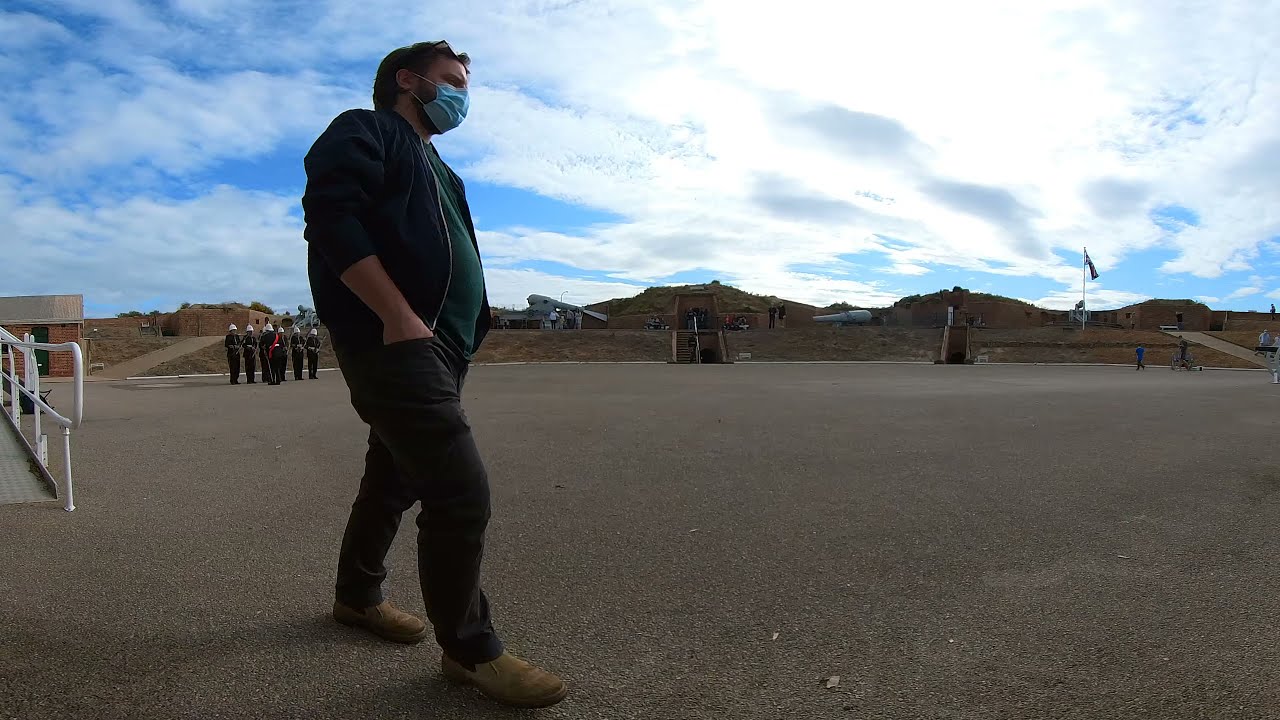In this outdoor image, a man wearing a blue surgical mask appears to be walking in what looks like a parking lot with a paved surface. He is donned in a black hooded sweatshirt with the zipper undone, revealing a green t-shirt underneath. He also wears black pants and brown boots, with his hands tucked into his pockets. The man has brown hair and looks to be in his early 30s. The sky is a mix of blue and white clouds, indicating a clear day with no impending bad weather, and the sun is peeking out from behind the clouds.

In the background, on the left side of the image, there is a steel ramp with a white handrail near a small brick building, suggesting a possible school or similar establishment. Further to the left, there's an incline with a pathway leading to another rectangular brown building, and nearby soldiers in black uniforms with white helmets are seen standing in formation. The front soldier appears to be holding or wearing something red.

The distant backdrop features a hilly landscape with several sets of concrete steps leading up the hill, possibly indicating a tiered terrain or constructed earthworks. Additionally, there is an American flag visible on the right side of the image, further enhancing the setting with a sense of institutional or ceremonial space.